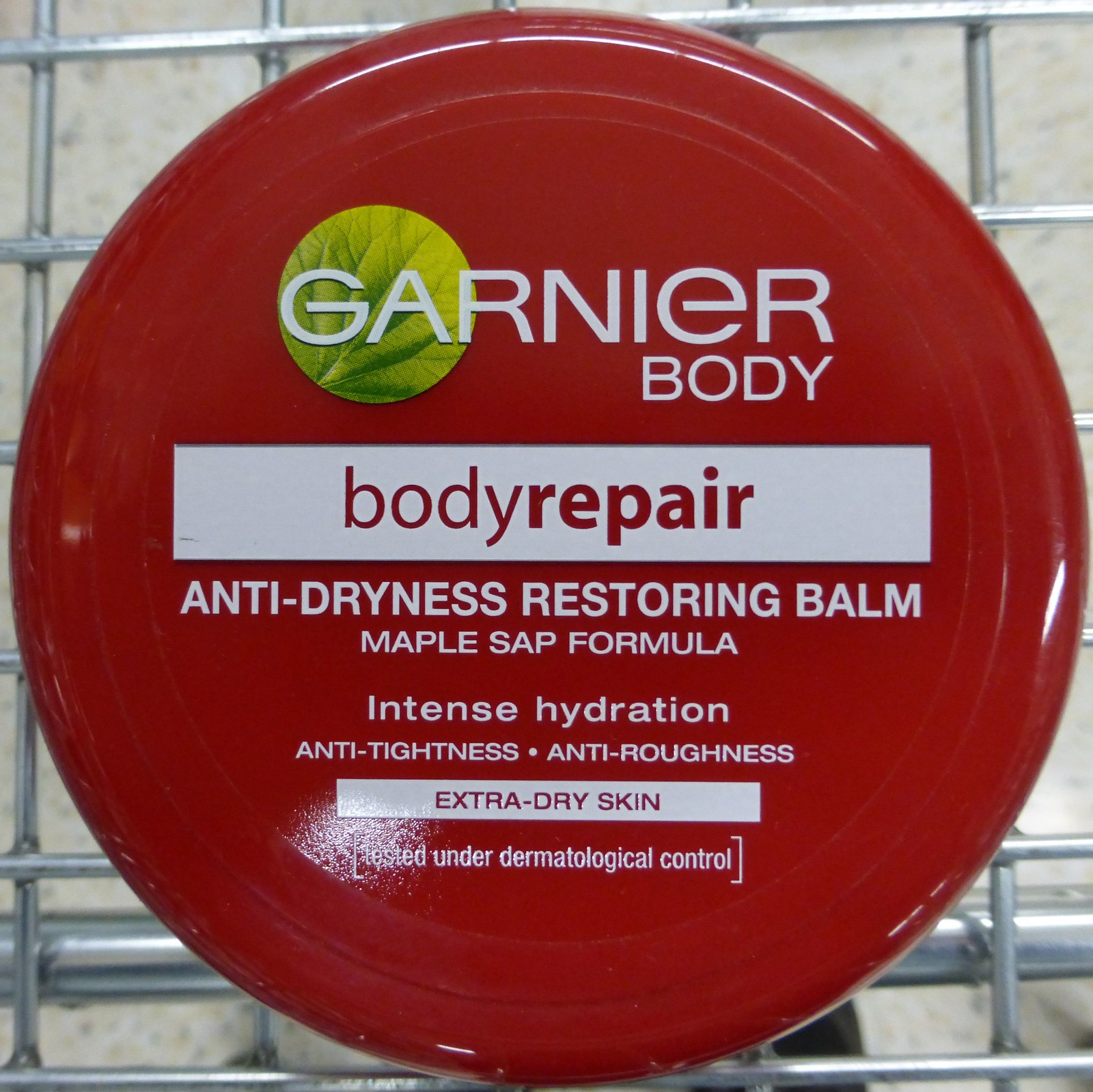This image features a top-down view of a red capped jar of Garnier Body Repair, captured likely from a shopping cart. The prominently red jar features detailed white text and a small green circle behind the "G" and "A" of Garnier which is textured like a leaf. The label includes "Body Repair" in red letters on a white background in the middle section, followed by "Anti-Dryness Restoring Balm," "Maple Sap Formula," "Intense Hydration," "Anti-Tightness," "Anti-Roughness," and "Extra Dry Skin" written on the red background below. The phrase "Tested under Dermatological Control" is also mentioned in smaller text. The context suggests a metallic wire grid background, indicative of a shopping environment, possibly chrome surfaces like those of a cart. The position of the feet further confirms that this product is likely still being purchased.